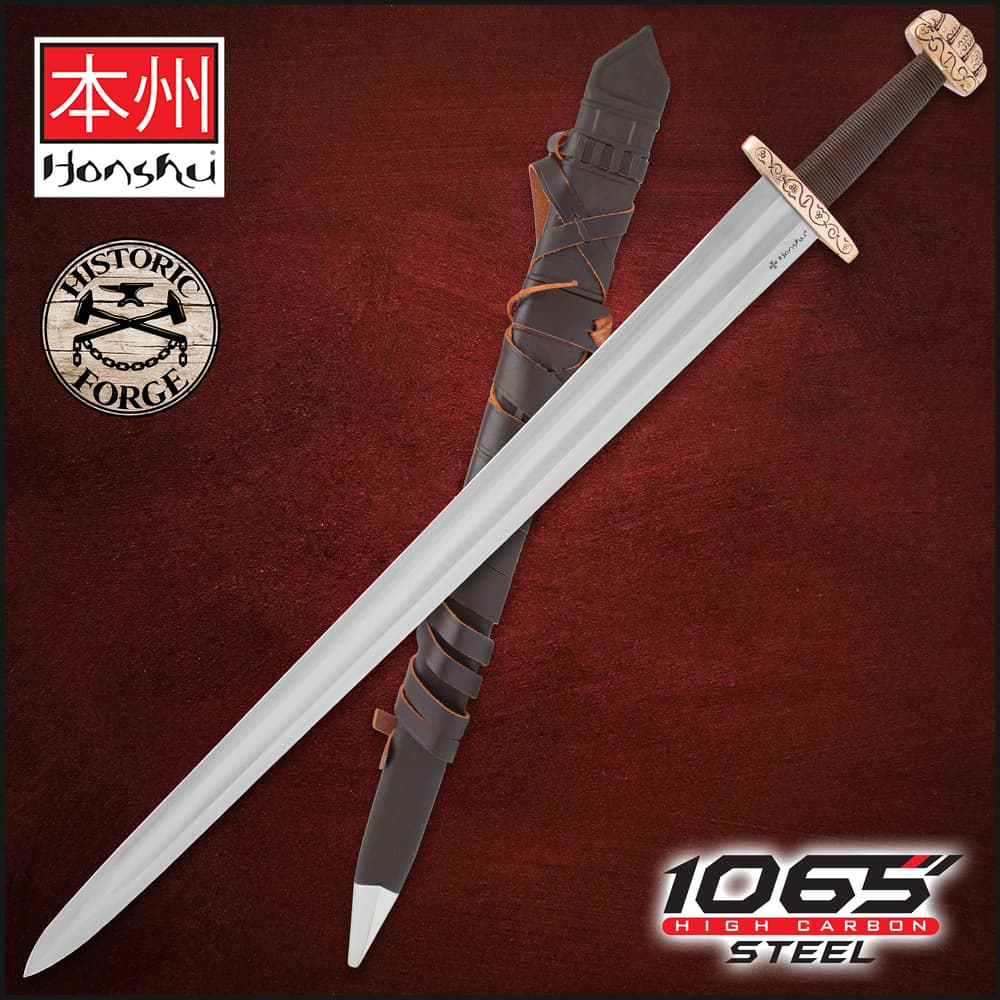This image is an advertisement for a sword featuring the brand "Honshu." Prominently displayed in the center, the long and smooth silver blade is angled diagonally from the top right to the bottom left. The sword boasts a detailed and ornate handle with a ribbed dark brown handgrip, complemented by carved gold or brass elements at both the hand protector (guard) and the pommel to prevent slippage.

In the top left corner of the image, a red square contains Japanese symbols in white, situated above a white square with "H-O-N-S-H-U" written in black letters. Nearby is a circular logo labeled "Historic Forge," featuring crossed hammers and an anvil set against a brown wooden background. 

Along the bottom part of the image, "1065 High Carbon Steel" is clearly mentioned, indicating the material quality of the blade. Additionally, the bottom right corner of the advertisement includes an inset picture depicting the sword sheathed in a leather scabbard, secured with brown straps and capped with a silver tip. This comprehensive layout highlights both the craftsmanship and the functionality of the Honshu sword.